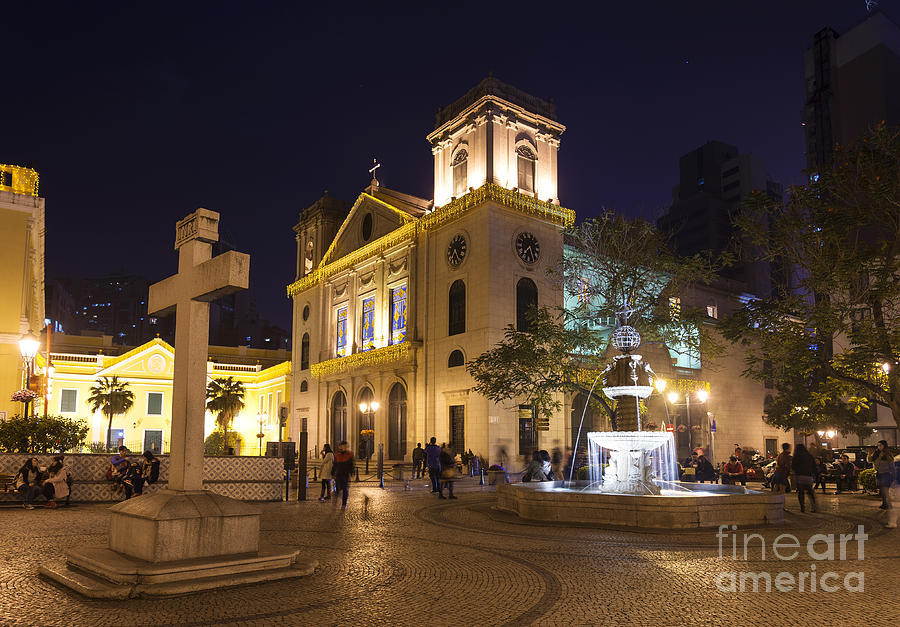This nighttime photograph from a web page titled "Fine Art America" captures a beautifully illuminated church courtyard. At the forefront stands an aged cement cross, appearing to have weathered centuries, positioned before the church entrance. To the right of the cross is a substantial water fountain with a decorative top, from which water actively flows down into a lower basin. The scene is teeming with architectural details; notably, the church itself has another cross atop its roof and an elaborate belfry-like structure rising from the right side. The building's grand second story features at least three stained glass windows, adding a touch of colorful elegance to the facade. Adjacent to the main church, another part of the building is distinctly painted yellow. The entire area is bustling with life, as people stroll through the well-lit plaza, creating a serene yet vibrant atmosphere.